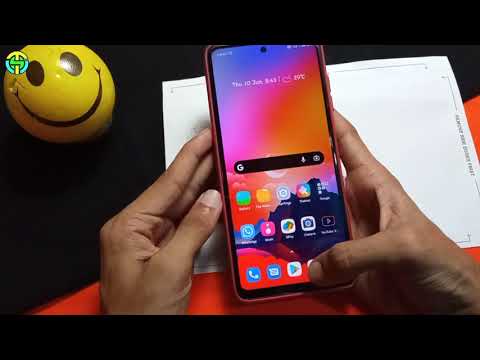The photograph showcases a pair of brown hands holding a smartphone with a vibrant red-to-blue gradient background image. The hands and phone rest on a flat surface, partially covered by a white sheet of paper. Below the paper, there's a red rectangular strip that angles from the bottom left to the upper right, splitting the backdrop into two triangles. The lower triangle includes the surface and paper, while the upper triangle is a stark black void. Notably, a three-dimensional yellow smiley face with large black eyes and an exaggerated smile occupies the upper left corner. The phone's colorful home screen boasts hues of blue, pink, orange, and red, with a Google search bar prominently displayed amidst various apps.